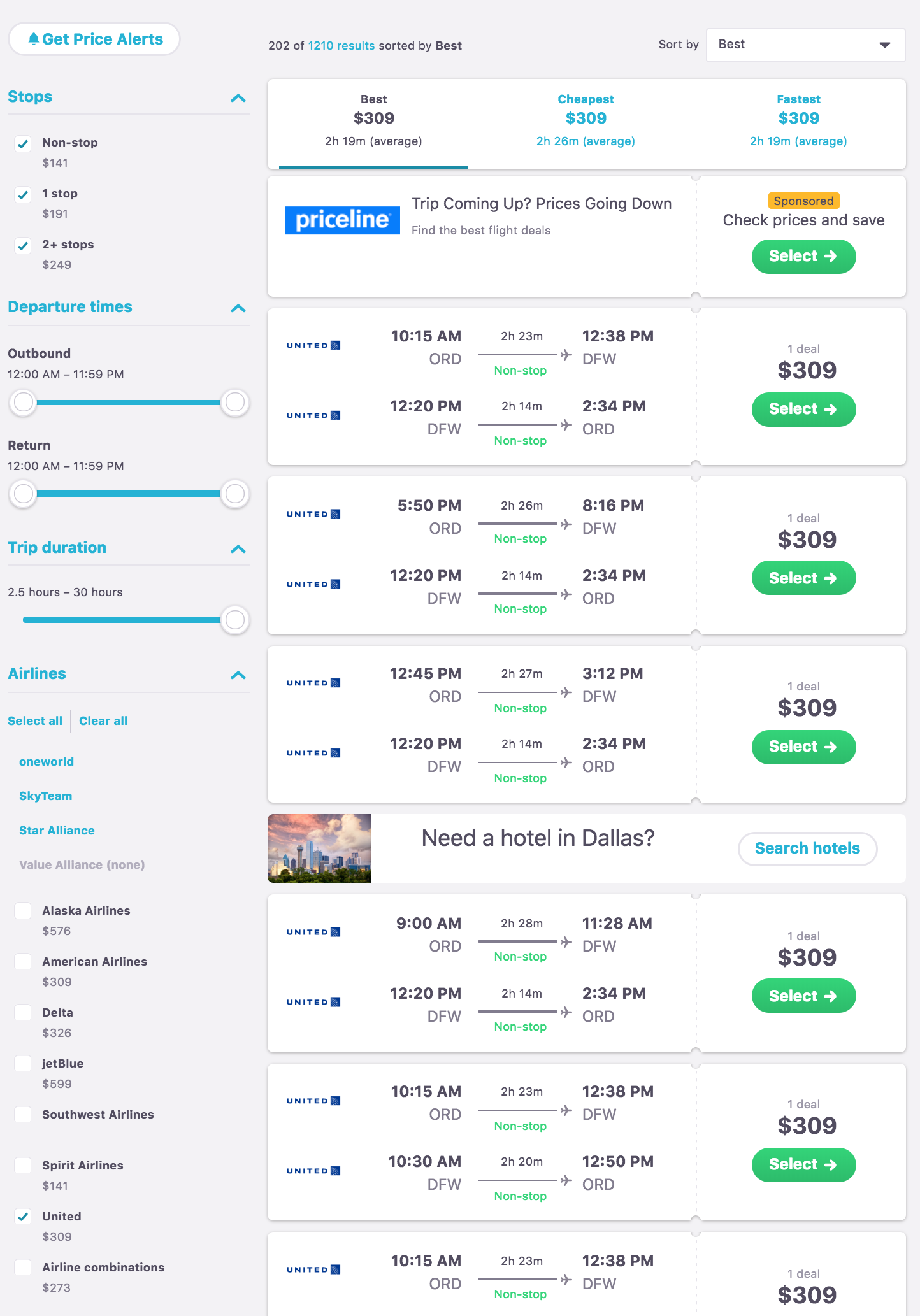The image depicts a detailed search interface for airline flights from Chicago to Dallas-Fort Worth and back. At the top of the interface, there is an option to enable price alerts, accompanied by a note stating "202 of 1,210 results sorted by Best" with a dropdown menu allowing different sorting preferences, currently set to "Best."

On the left side of the interface, filtering options are listed:

1. **Stops:** Checkboxes are marked for non-stop, one stop, and two-plus stops.
2. **Departure Times:** Sliders indicate the selected outbound and return times, both set between 12 a.m. and 11:59 p.m.
3. **Trip Duration:** Another slider allows selection of the trip length, currently set between 2.5 hours and 30 hours.
4. **Airlines:** A section where all or specific airlines can be selected or cleared. Options include:
   - Alliances: One World, SkyTeam, Star Alliance
   - Airlines: Alaska Airlines, American Airlines, Delta, JetBlue, Southwest Airlines, Spirit Airlines, United Airlines, and Airline Combinations. United Airlines is marked with a green check mark.

On the right side of the interface, flight options are displayed, sorted by criteria such as "Best," "Cheapest," and "Fastest," each accompanied by their respective prices. Below each flight's cost, a green "Select" button with a white arrow is available for booking the desired flight. The listed flight details include departure and arrival times, prices, and layover information, providing a comprehensive comparison for the user.